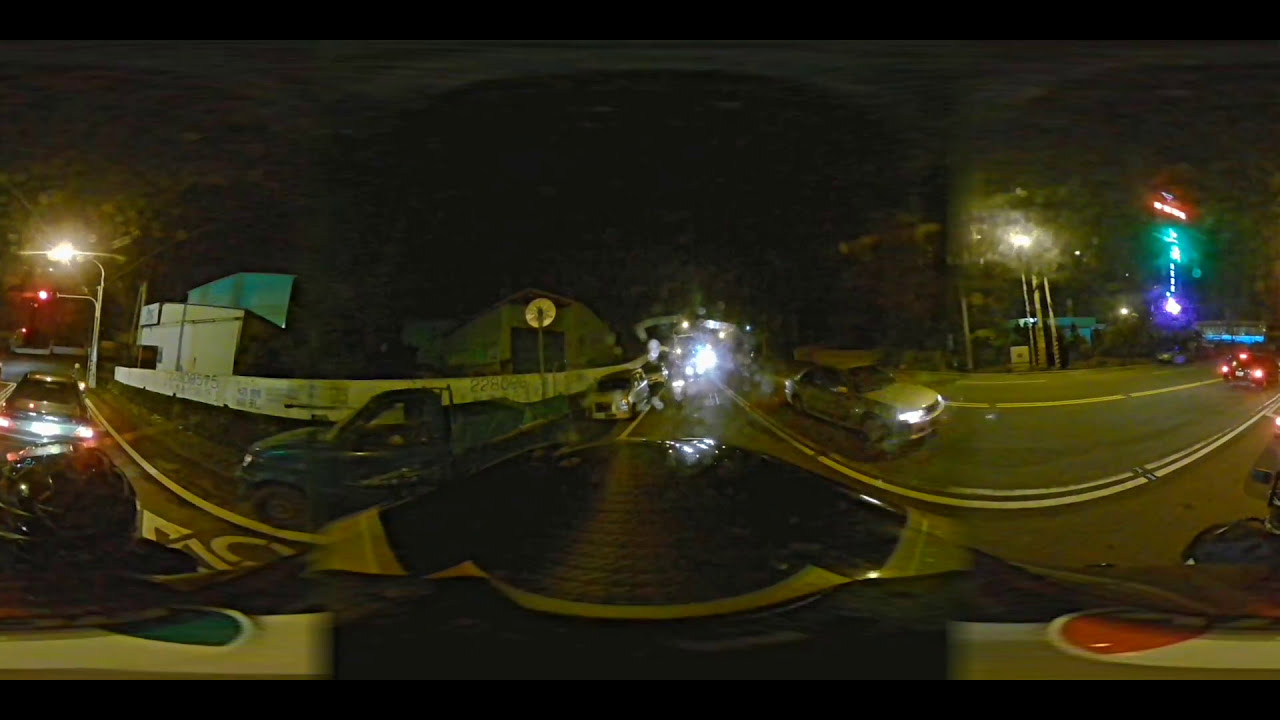The image depicts a nighttime urban scene captured from a high vantage point, likely from a semi-truck tractor trailer, as it navigates a bustling city street. The curvature of the ocular lens creates a panoramic view. The vehicle, which has white handlebars with green and red buttons, is moving down a multi-lane road. Cars are driving in both directions, adding to the busy atmosphere.

To the left, there is a red traffic light illuminating the street, in front of which a car with its red brake lights is stopped. Diagonally behind this car, there is a smaller, dark blue truck with its lights off, followed by three parked cars. On the right side of the image, there's a black car with three distinct red lights and, adjacent to it, a building adorned with signs in blue, red, and neon bluish-green. Another vehicle, a white coupe with its white lights on, is parked further along. 

Additionally, a gas station and a store with a sign partially obscured by a tree are visible on the right corner. Various other lights and traffic signs dot the scene, contributing to the overall brightness despite the nighttime setting. The road seems busy, with multiple cars moving in both directions, some heading straight towards the viewer.